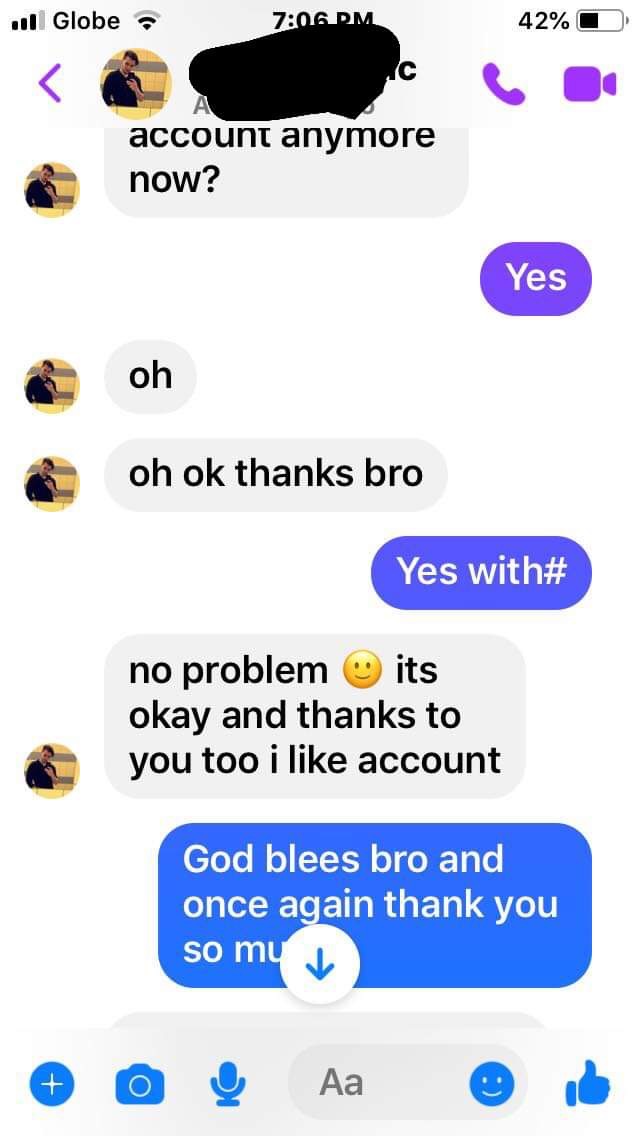The image is a detailed screenshot of a smartphone conversation within a texting app. At the upper left corner of the screen, there are three out of four mobile data bars filled, next to the word "globe". In the middle, the time reads 7:06 p.m., and on the right, the battery is at 42%. The names of the individuals involved in the conversation are blacked out. 

The message thread includes a series of text exchanges: 
- Person A: "Account anymore now?"
- Person B: "Yes."
- Person A: "Oh, okay, thanks, bro."
- Person B: "Yes." (accompanied by a hashtag symbol)
- Person A: "No problem😊, it's okay, and thanks to you too, I like account."
- Person B: "God bless, bro, and once again, thank you so much." (with the word "bless" misspelled as "blees")

At the bottom of the screen, standard icons for adding images, voice-to-text, typing a message, smiley emoji, and thumbs up are visible. The design elements include purple and gray chat bubbles, with some icons highlighted in blue.